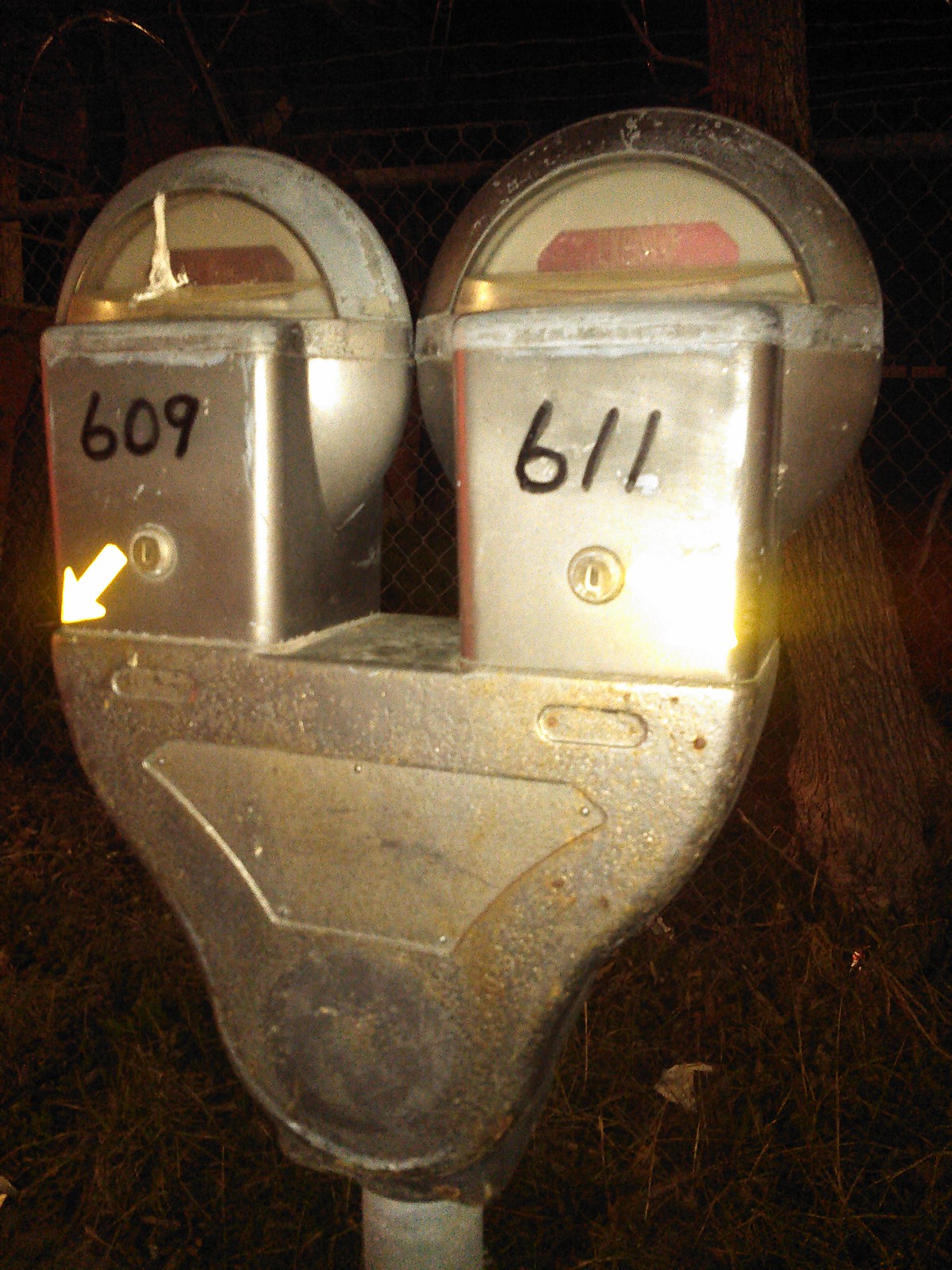The photo captures a double, silver, old-fashioned parking meter situated at night, illuminated by a flash. The meters are mounted on a single pole and are notably worn, dingy, and dirty. Both meters are expired, indicated by their red blinkers. The left meter displays the number "609" in black marker, while the right one shows "611". A distinctive feature is the small yellow arrow pointing southwest at the bottom of the "609" meter. The left meter is marred by bird droppings on its clear time display.

In the background, a dimly lit scene reveals a chain-link fence topped with barbed wire and a leafless tree to the right. Ground-level details include dark brownish-green shrubs and twigs. The overall setting is dark, with camera glare visible near the base where the meters connect to the square mounting pole.